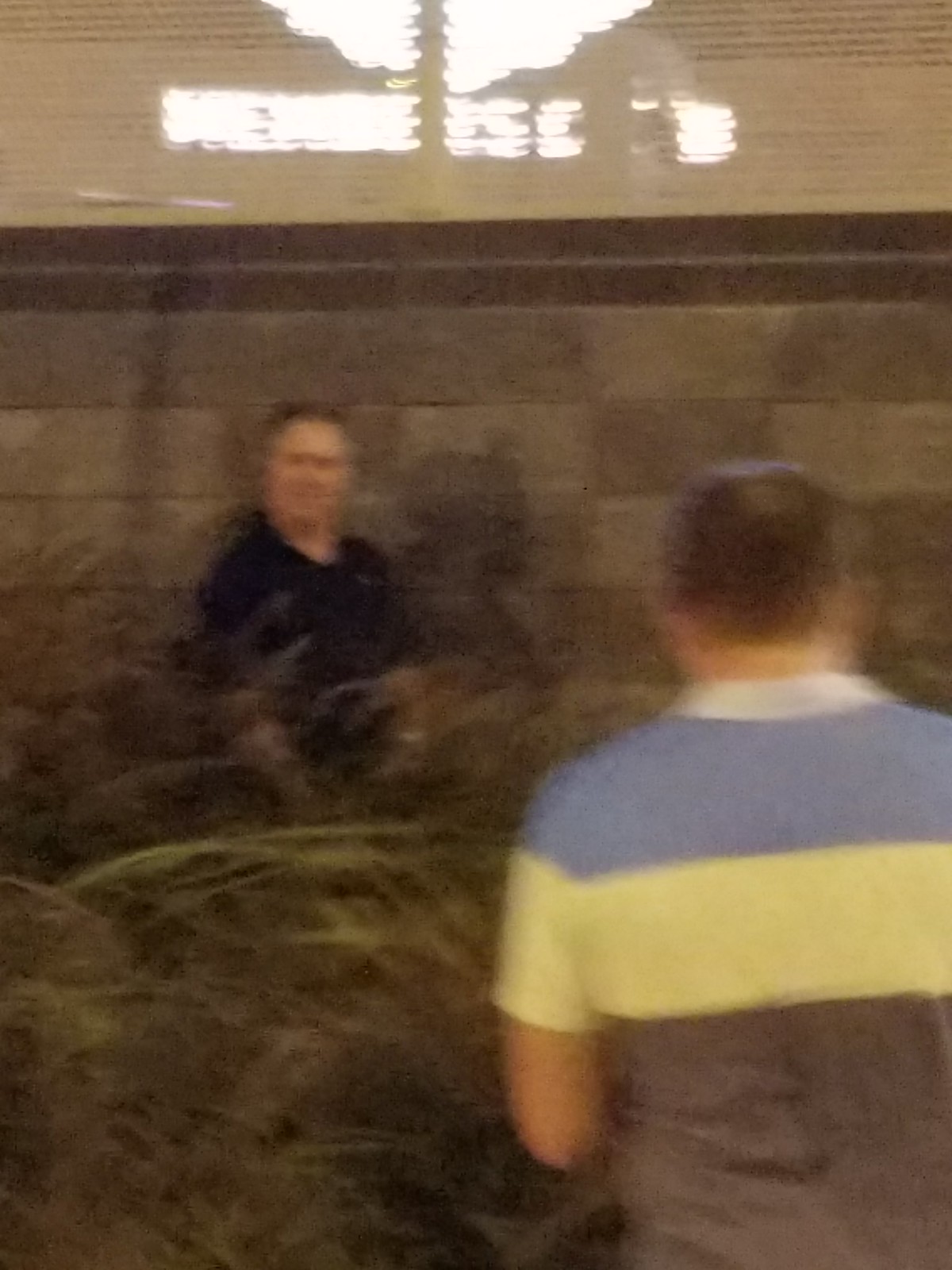The photograph depicts an individual dressed in a tri-color polo shirt intently gazing at a man who appears to be either a cashier or a receptionist. The setting suggests a bustling environment, likely a casino, as evidenced by the blurred background featuring vibrant lights and gaming machines. The composition captures a moment of interaction, highlighting the anticipation or curiosity of the polo-shirted person while the worker remains focused on their task.